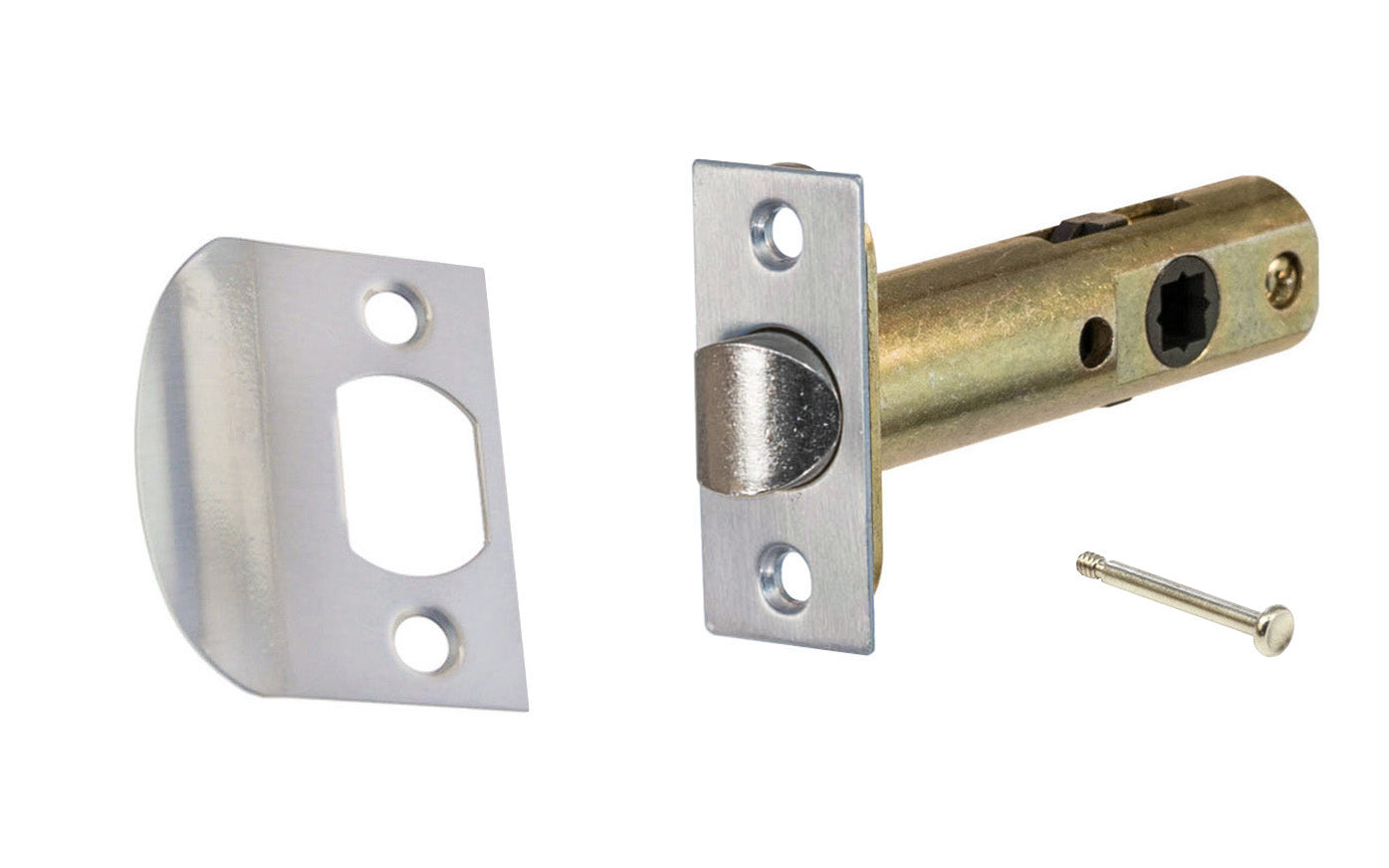This image depicts the components of a door lock mechanism, showcasing both the strike plate and the latch. The scene is set against a white background. On the left side of the image, there is a vertical, rectangular, silver strike plate featuring three holes: one at the top, one at the bottom, and a larger, rounded square opening in the middle. Lying at the bottom is a bright silver screw with a threaded tip, indicating it is used for fastening. Adjacent to the strike plate is the latch mechanism, which consists of a gold or copper-colored cylindrical section and a silver front plate. The front plate has two small holes for screws and a centralized protruding latch piece designed to fit into the corresponding middle opening on the strike plate. The intricate details of the metal parts and their specific arrangements suggest this is a complete door locking system, including elements used to securely attach it to a door frame.